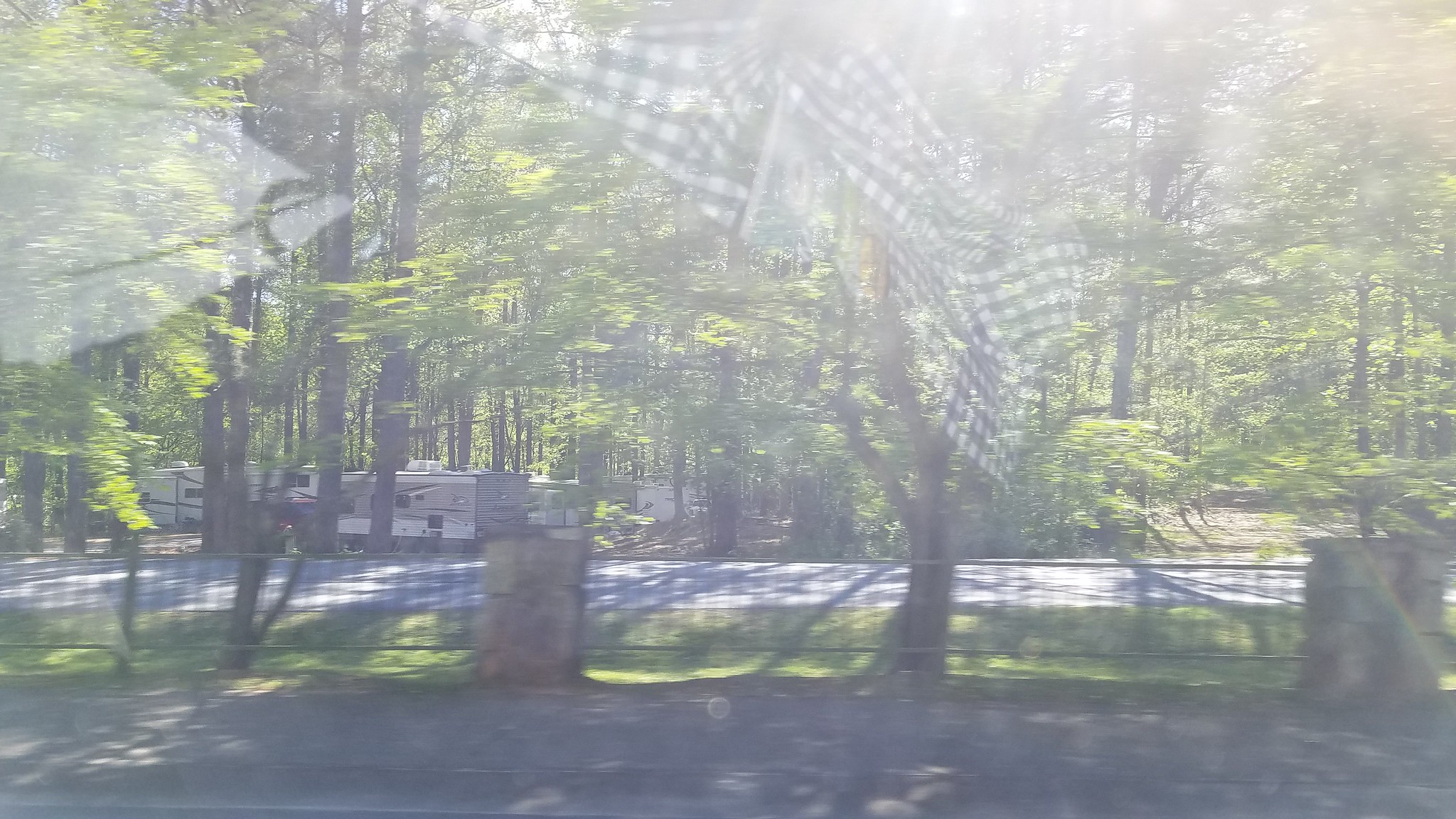This slightly blurry photograph, likely taken from a moving vehicle on a sunny, windy day, captures an outdoor scene of a campground or rest area. The motion and sunlight create a slight reflection in the image, reinforcing the sense of movement. The foreground features a well-maintained asphalt road bordered by a black wrought iron fence with brownstone or rock columns dotting the fence line. Behind the fence lies a grassy area leading to a heavily wooded section with tall trees that appear to be swaying in the wind. On the left-hand side of the photograph, several white and beige trailers or RVs are parked in what looks to be a trailer park or campground, providing a resting place for travelers. The sun, likely positioned at midday or late afternoon, bathes the entire area in light, casting soft shadows and illuminating the green leaves and brown tree trunks. The bottom portion of the photo shows patches of brown dirt, completing the rustic outdoor setting.